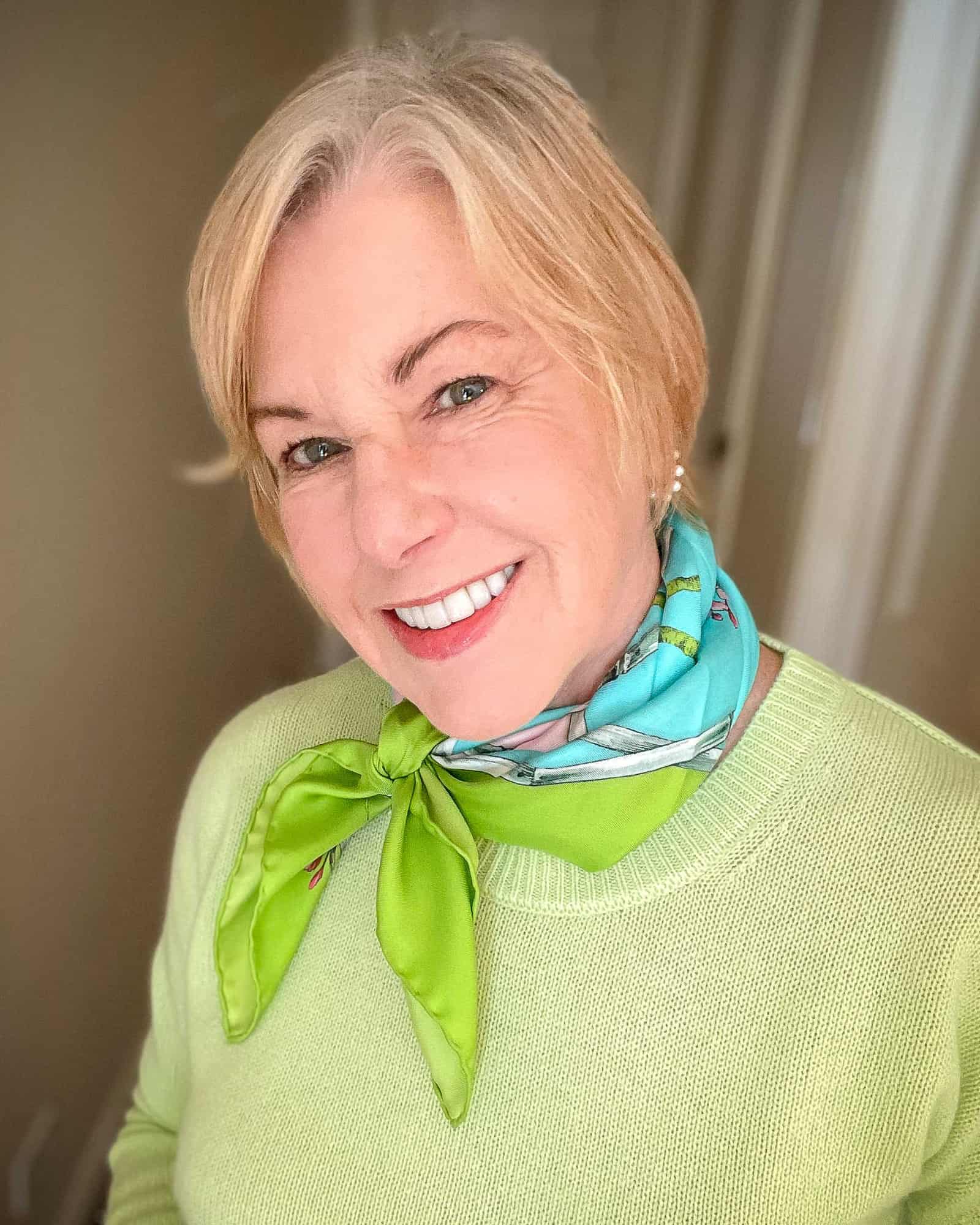This close-up photograph features a friendly woman, smiling sweetly at the camera. She appears to be in her 50s or early 60s, with well-cared-for skin. Her short, ear-length blonde hair is neatly pulled back, revealing small pearl earrings peeking through. Her blue or bluish-gray eyes are framed by beautifully arched eyebrows. She wears light makeup, including lightly applied red lipstick, and shows off her straight, white teeth.

Around her neck is a vibrant silk scarf, predominantly light blue and lime green, with a delicate design pattern. It ties into a cute bow, complementing her scoop-neck, knitted lime green sweater. The background features a beige wall on the left and sheer, light-colored curtains, slightly blurred to keep the focus on her warm, inviting expression.